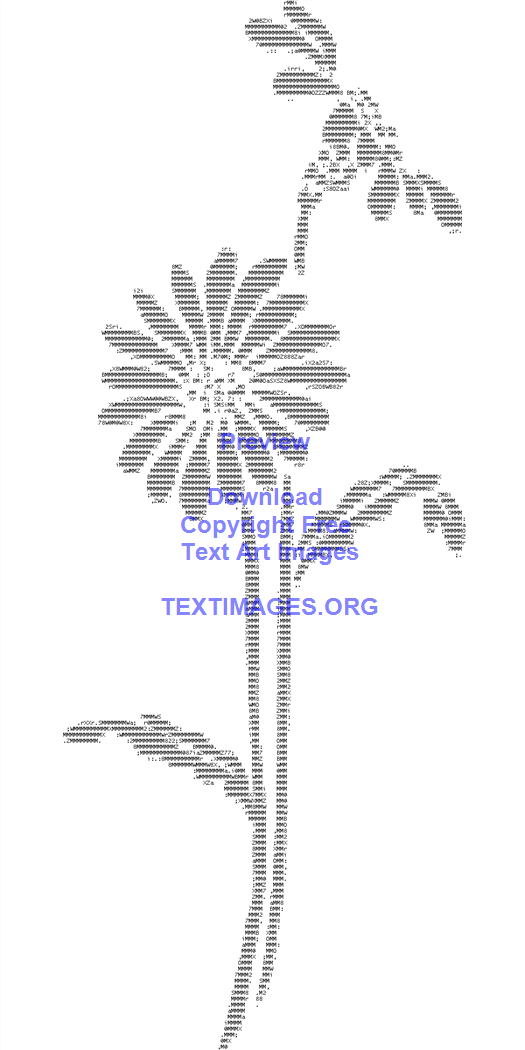This image showcases a detailed black and white clip art-style flower illustration created using text characters, though the characters themselves are too small to identify. The image consists of two flowers, each with a long stem and one leaf. The taller flower, which leans to the right, is viewed from the side, revealing its slender profile. The shorter flower, facing forward, displays its petals more clearly. The background is stark white, accentuating the intricate text art design of the flowers. Adding a splash of color, blue text overlays the center of the image, reading "Preview. Download copyright free text art images. textimages.org," serving as a watermark. This text is the only colored element in the otherwise monochromatic artwork. The impressively detailed composition highlights the creative use of keyboard characters to form shapes and patterns, emphasizing the artistry involved in crafting this piece.